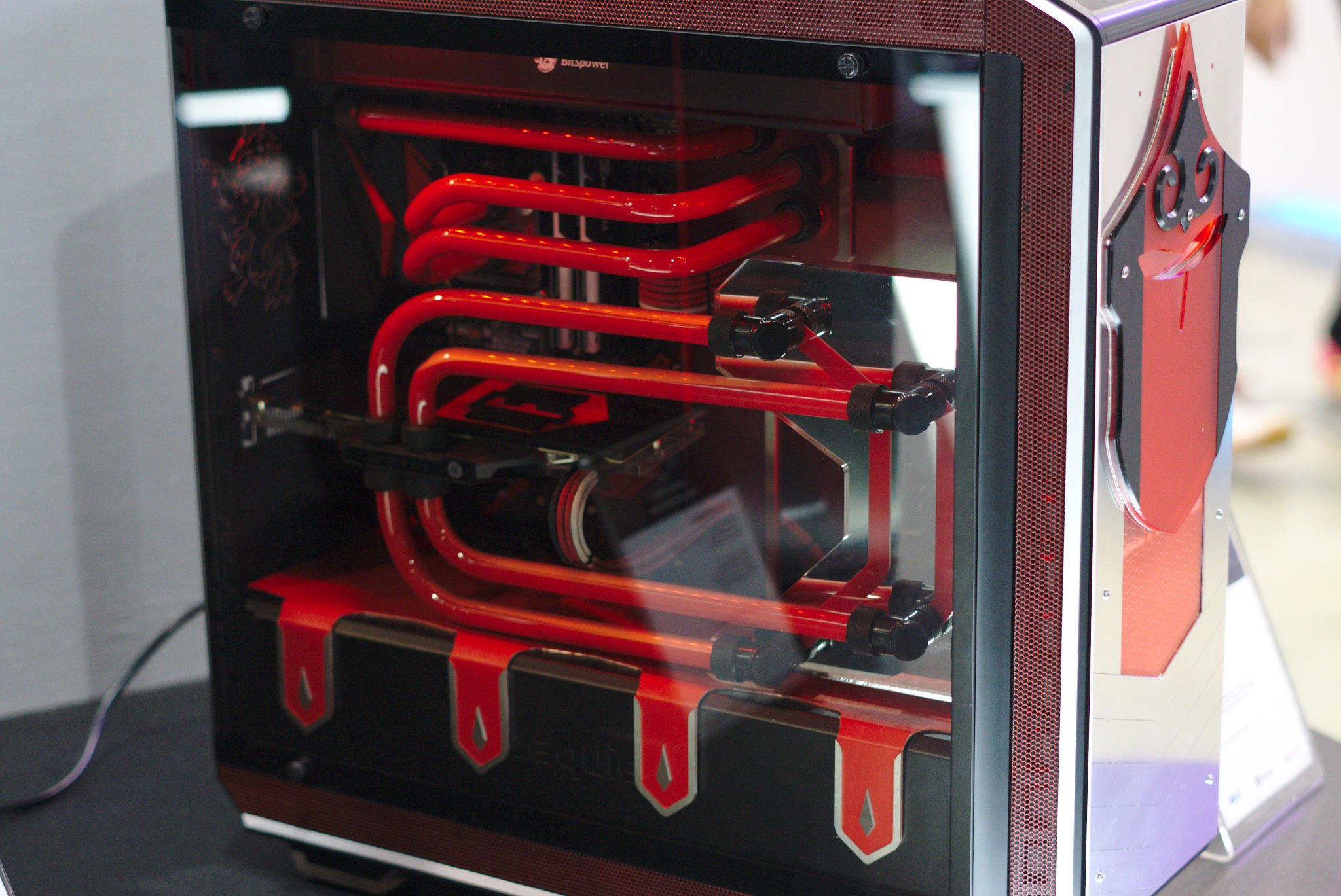The image depicts a sleek, tower-based personal computer featuring a transparent left-side panel that reveals an intricate liquid-cooling system. The machine prominently displays red, curved tubes that snake throughout its interior, connected by black segments, resembling coiled cords. These tubes are designed for efficient cooling, particularly past the CPU, hinting at high-performance capability, as indicated by the inscription "BitsPower" at the top. The computer case itself is a striking combination of black, silver, and red colors, with a notable design element on the front—a red background adorned with a black fleur-de-lis emblem and diamond-shaped motifs on the sides. Additional text inscribed at the bottom spells out "BEQIE." The entire setup is situated on a table, and the background of the image is deliberately blurred, drawing full attention to the sophisticated and visually detailed computer.